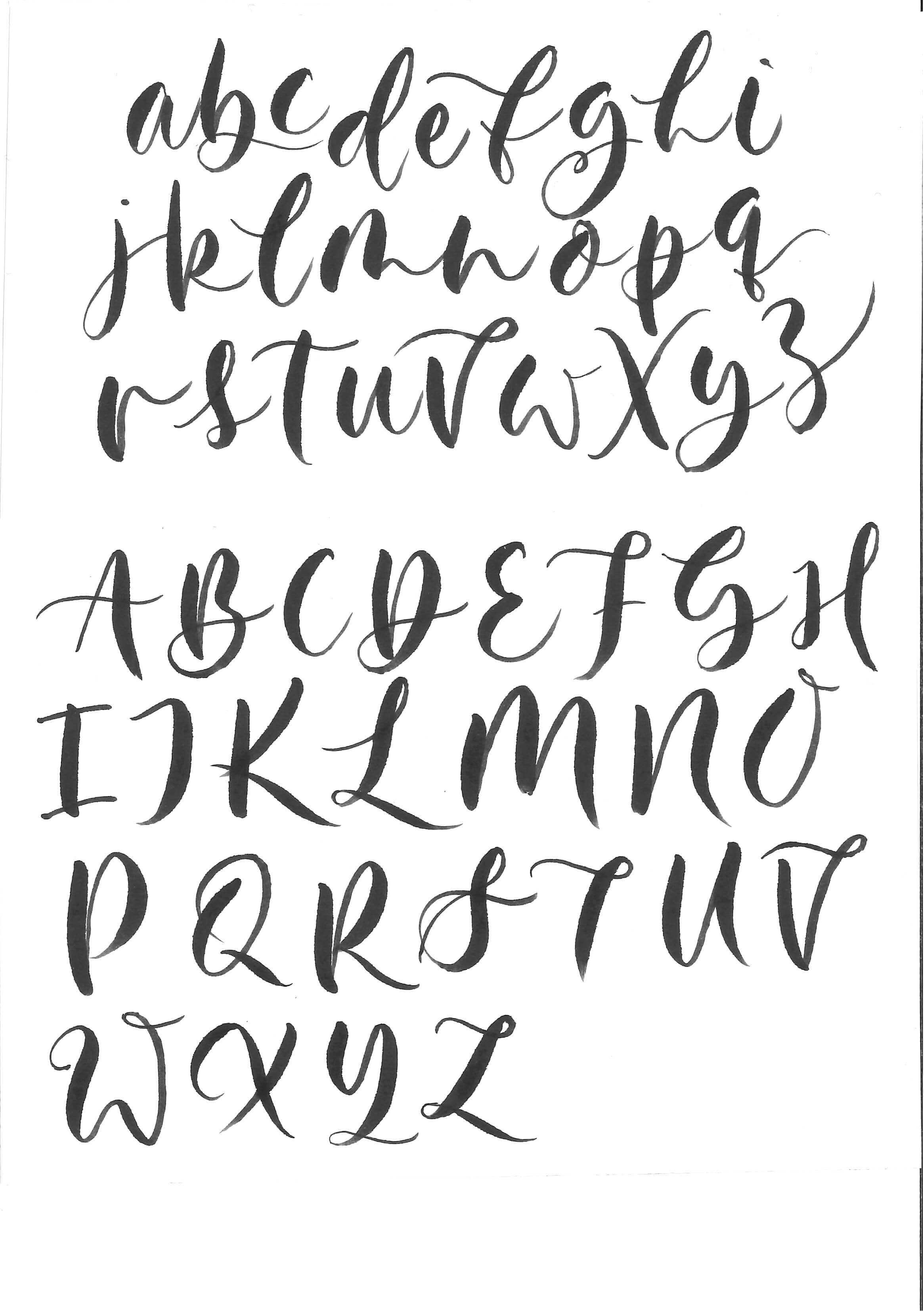This image displays a carefully crafted poster featuring the entire English alphabet in a specific type of cursive font, characterized by thick, stylized, and swoopy letters. The poster is laid out on a white background that resembles parchment paper, giving it a simple yet elegant look. The alphabet is presented in both lowercase and uppercase letters. The lowercase letters are arranged in three rows: the first row runs from 'a' to 'i', the second from 'j' to 'q', and the third from 'r' to 'z'. Notably, several lowercase letters are connected, such as 'a' and 'b' and 'j' and 'k'. The uppercase letters follow below in a similar three-row format: 'A' to 'H' in the first row, 'I' to 'O' in the second, and 'P' to 'Z' spanning across the last two rows, with 'W', 'X', 'Y', and 'Z' occupying the final spaces. The cursive script employs a dark gray color, resembling watercolor or calligraphy ink, with some sections of the strokes being thicker than others. A thin black line runs vertically along the right side, becoming slightly thicker towards the bottom, adding an accent to the overall minimalist design and emphasizing the vertical layout. The poster maintains balanced white space, providing a clean and uncluttered appearance.